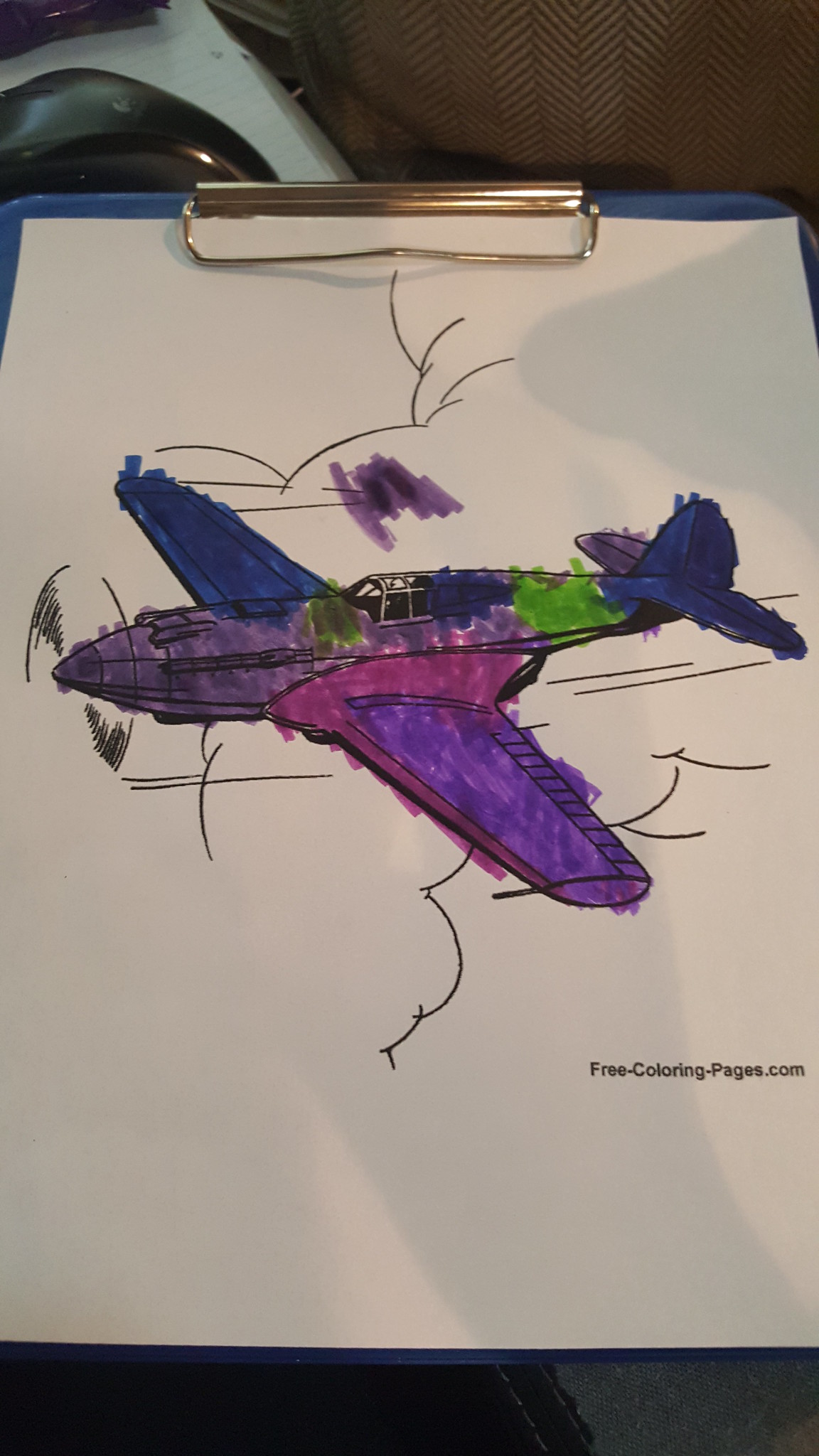This photograph showcases a coloring book page sourced from FreeColoringPages.com, as indicated by the website's URL written in black ink at the lower right corner. Printed on standard white printer paper, the page features an image of what appears to be a fighter plane, potentially from a historical war era. The plane is vividly colored using markers, evident from the overlapping lines that create darker, choppier edges.

The wings of the plane display an eclectic mix of purple, pink, and blue hues, while the body combines shades of pink and purple, accented with green and blue towards the tail. The plane, depicted soaring through the sky, is surrounded by stylized clouds, some delineated in black and white, enhancing the scene's dynamic nature.

The coloring page is affixed to a clipboard, suggesting it is positioned on a flat surface such as a table or chair, though it could also be resting in a more unconventional setting like the interior of a car. The overall presentation reveals the playful and creative effort put into bringing the plane to life with vibrant colors.